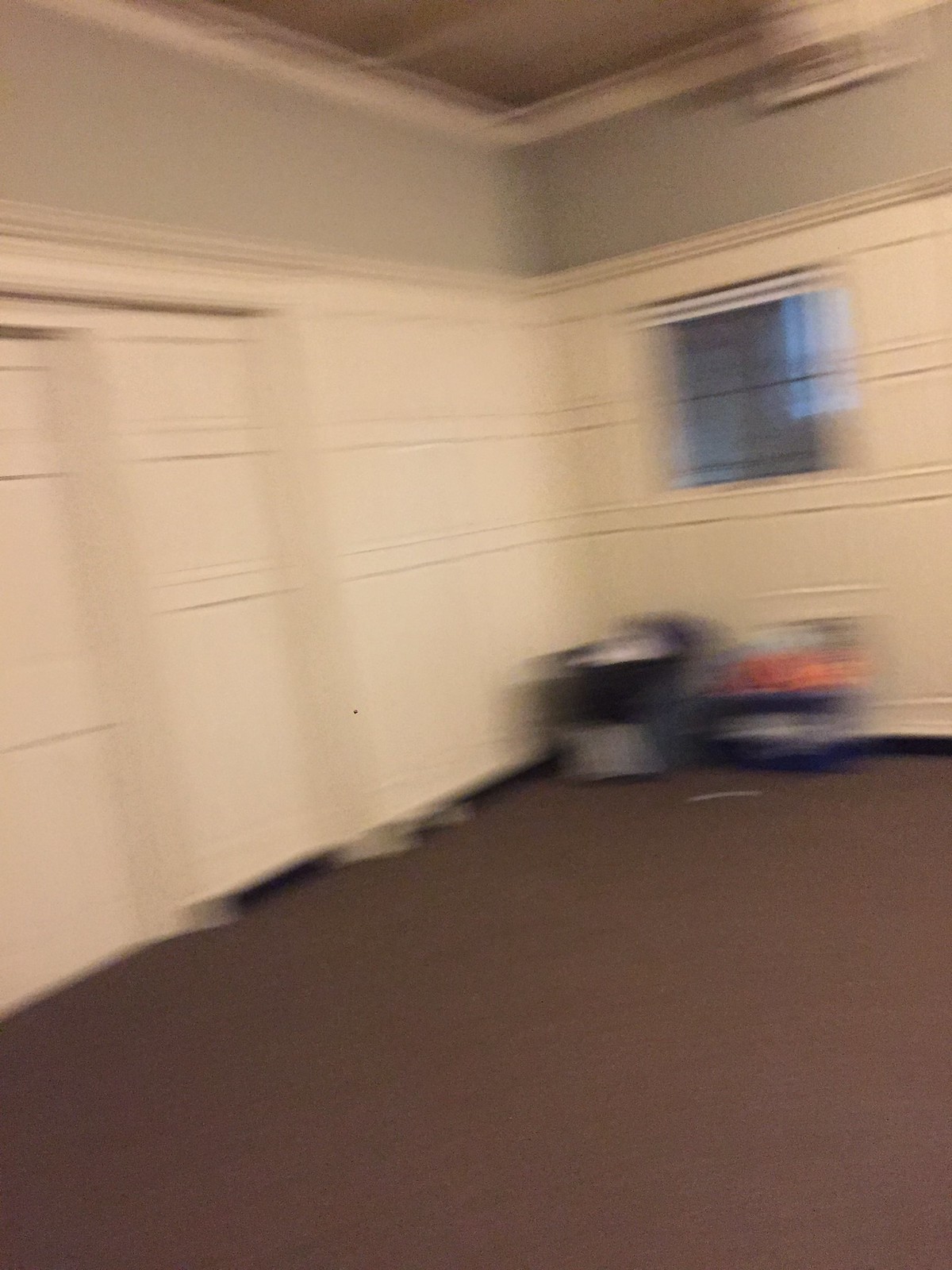This photograph captures the interior of a nondescript room, albeit with a significant amount of blur, suggesting movement during the shot. The room features predominantly white walls: one on the left and another directly ahead. A small, basement-like window is visible on the forward-facing wall, which allows minimal natural light into the space.

In the distance, two metallic objects can be discerned. One resembles a silver trash can, while the other appears to be another silver appliance or device, though its specific function is unclear. The floor is unremarkable, covered in a dark brown surface that adds to the room's utilitarian feel.

Above the white walls, there is a strip of gray-painted wall on both sides, providing a subtle contrast. The ceiling is partially visible, showing a mix of brown and white tones. Despite its simplicity, the room's functional elements and the photography's motion blur add a layer of intrigue to its otherwise mundane appearance.